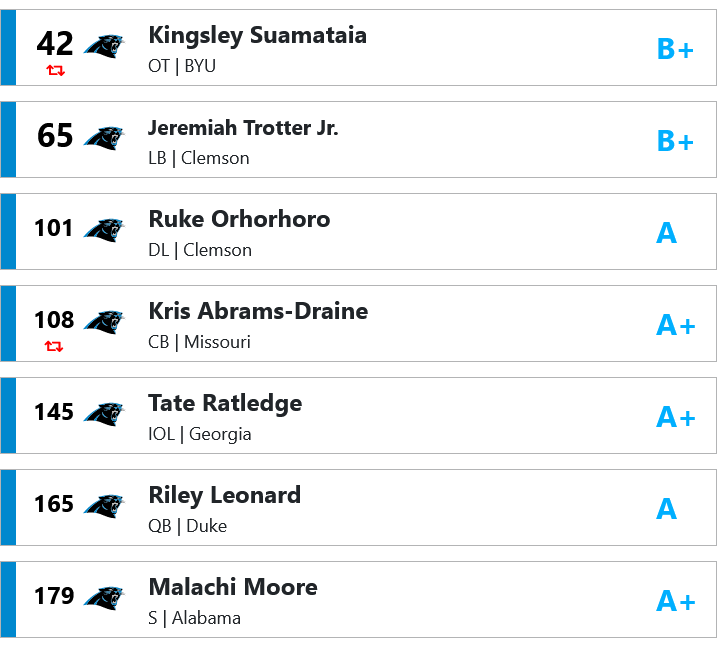The image is a screenshot featuring a list of various football players against a white background. The overall shape of the image is slightly taller than it is wide. It consists of several long, horizontal rectangles stacked on top of each other, with a small white space separating each rectangle. 

Each rectangle has a distinct design: a vertical royal blue strip on the left side, followed by a blue gradient bar on the right side. Inside each rectangle, there is a sequence of elements presented in a precise manner. From left to right, each rectangle contains:

1. A number.
2. A logo featuring a black panther, likely representing the Carolina Panthers.
3. The player's name in bold.
4. The player’s position, abbreviated.
5. The University the player came from.
6. A grade assigned to the player.

The players listed from top to bottom are as follows:

1. Number 42: Kingsley Suamataia, OT, BYU, Grade: B+
2. Number 65: Jeremiah Trotter Jr., LB, Clemson, Grade: B+
3. Number 101: Ruke Orhorhoro, DL, Clemson, Grade: A
4. Number 108: Kris Abrams-Draine, CB, Missouri, Grade: A+
5. Number 145: Tate Ratledge, IOL, Georgia, Grade: A+
6. Number 165: Riley Leonard, QB, Duke, Grade: A
7. Number 179: Malachi Moore, S, Alabama, Grade: A+

This structured format provides clear and concise information about each player, their position, their university, and an evaluation of their skills through grades.